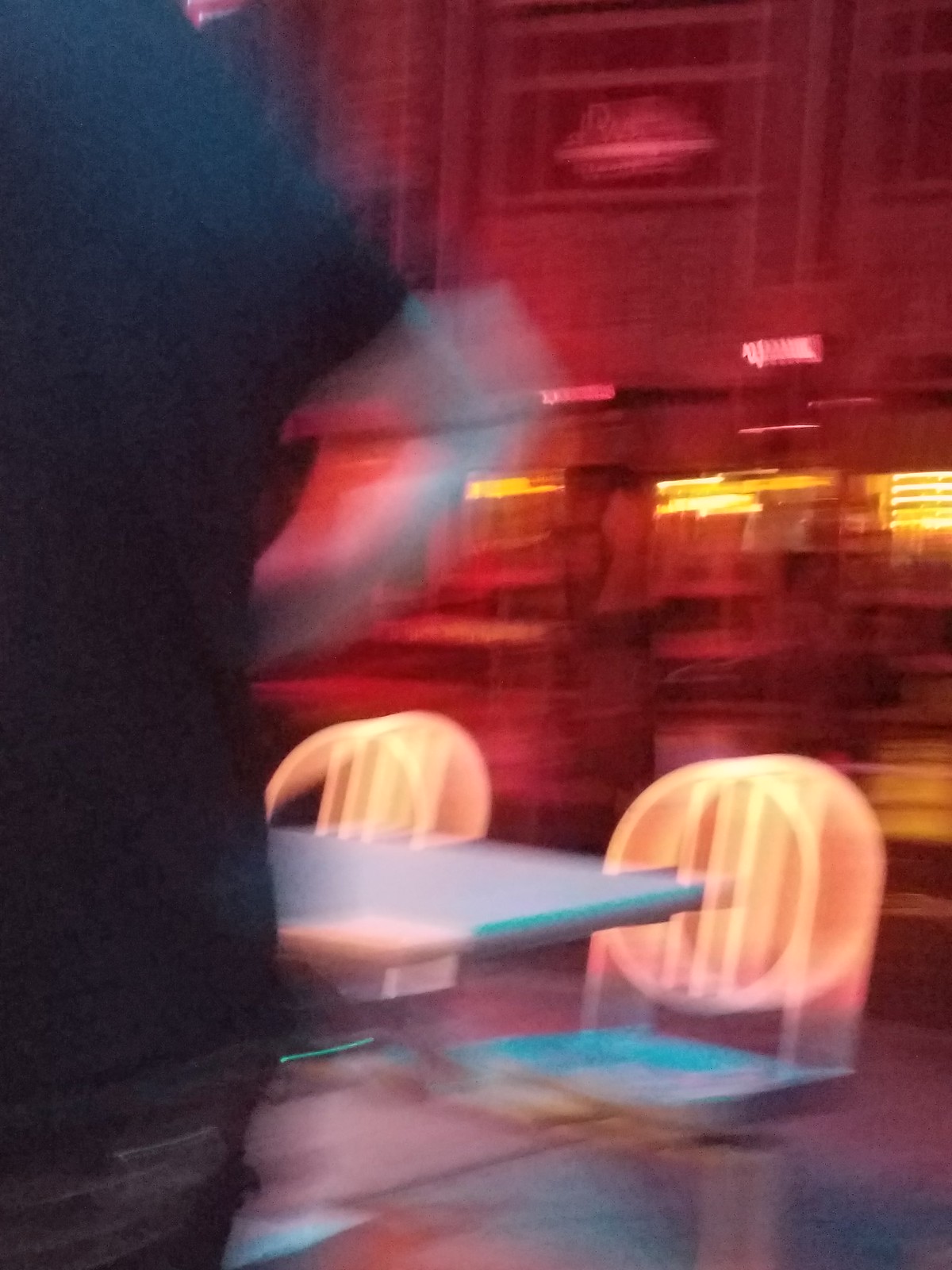This image captures a low-quality, blurry scene taken inside a building at nighttime. The dominant hues are red, with shiny and yellow lights creating a vibrant, albeit unclear, atmosphere. The top right corner features a lit-up yet unreadable sign. A person's back, donned in a blue shirt and blue jeans, occupies the entire left third of the photo, extending from top to bottom. Their pale, tan arm is bent at the elbow, suggesting motion. Below the figure, there is a small seating arrangement resembling a sidewalk cafe setup, featuring a blue table flanked by white chairs with yellow back braces. In the background, a road and storefronts are just barely discernible.